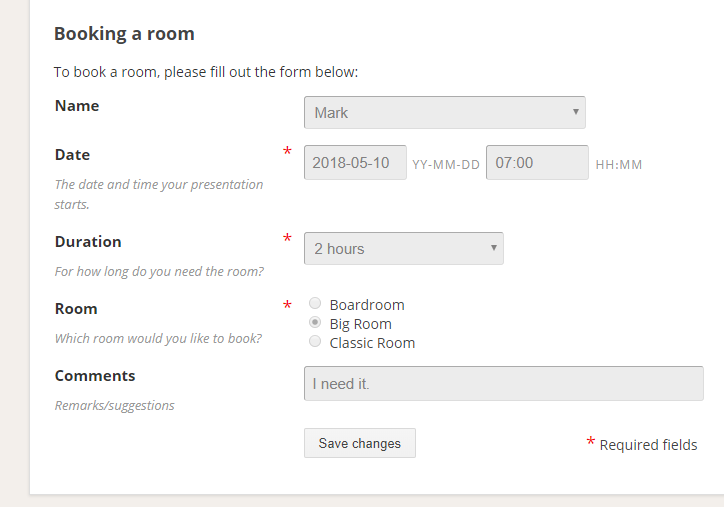This image is a zoomed-in screenshot of an online room booking form. Due to the zoom, some parts of the form appear to be cut off. The top of the form is labeled "Booking a Room" with a subheading "To book a room please fill out the form below." The form includes several fields:

1. **Name:** A text box where the name "Mark" is currently entered.
2. **Date and Time:** A required field (indicated by a red asterisk) where users input the start date and time of their booking. The format specified is "YYYY-MM-DD" for the date and "HHMM" for the time, with the current entry set to "2018-05-10" and "1900" (7:00 PM).
3. **Duration:** Another required field where the duration of the room booking is specified. This field is filled with "2 hours."
4. **Room:** A selection field for choosing the type of room to book, also marked with a red asterisk. The options available are "Boardroom," "Big Room," and "Classic Room," with "Big Room" currently selected.
5. **Comments, Remarks, Suggestions:** A text box for any additional comments, which currently contains the sentence "I need it."
6. **Required Fields Note:** At the bottom right, a message notes that fields marked with a red asterisk are required.
7. **Save Changes Button:** A button labeled "Save Changes" is located at the bottom of the form.

This form is designed to streamline the process of booking a room by clearly outlining all necessary information and required fields.